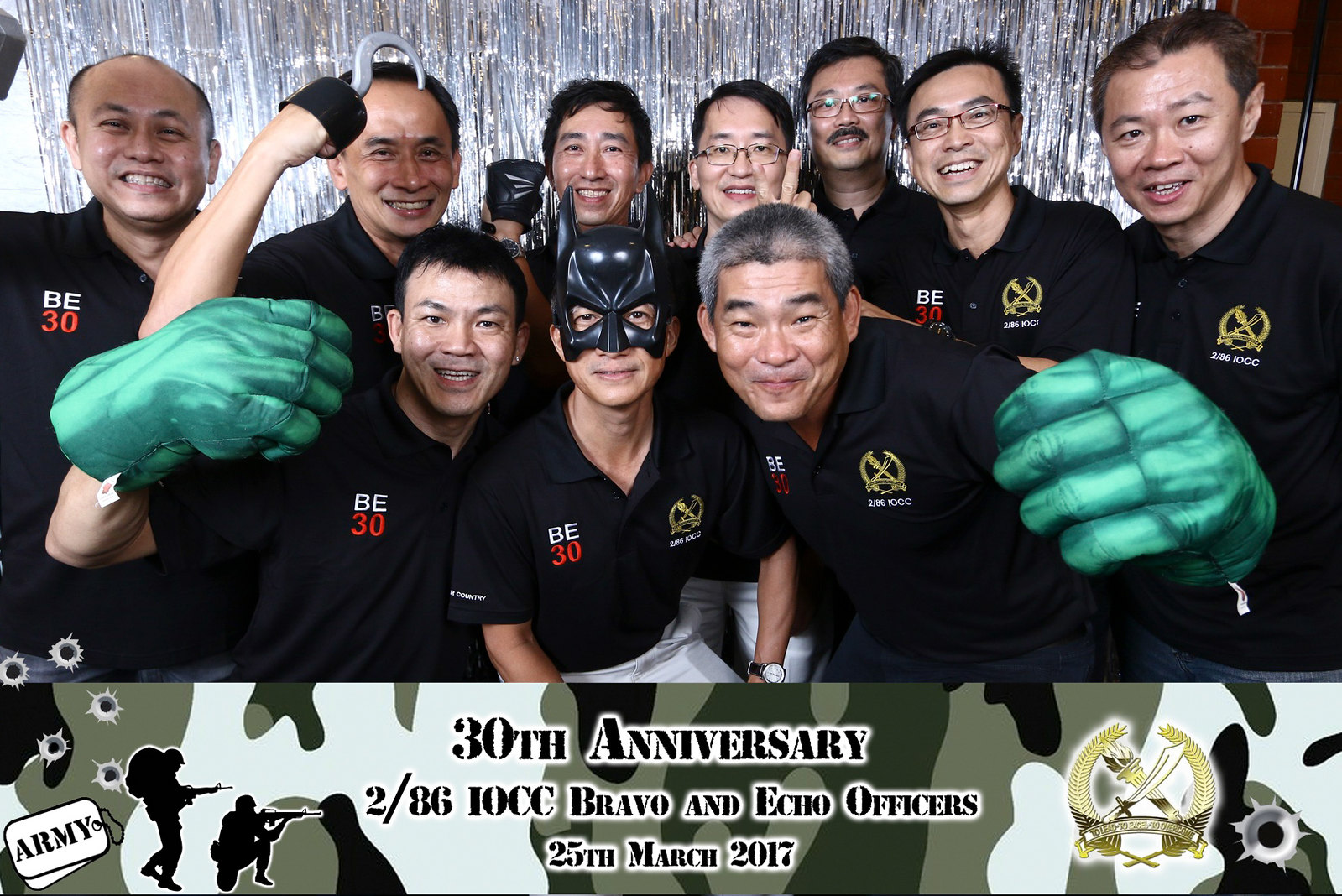In this landscape-mode image celebrating the 30th anniversary of the 2-86 IOCC Bravo and Echo Officers on 25th March 2017, a group of ten Asian men poses for a photograph, all smiling warmly. They are organized in two rows against a backdrop of silver and gold streamers. Each man is dressed in a black short-sleeved polo shirt featuring a white "B.E." emblem and the number "30" in red on the left chest. The central figure stands out by wearing a plastic Batman cowl, adding a playful touch to the scene. Flanking him, two men are each wearing a single green Hulk glove, while another man in the back row sports a pirate hook on his hand. In the lower quarter of the image, a camouflage-patterned banner bears the inscription, "30th Anniversary, 2-86 IOCC, Bravo and Echo Officers, 25th of March, 2017." To the left, the banner includes black silhouettes of army figures, bullet holes, an "Army" dog tag, and a small sign tagged "Army." On the right, there's a shield featuring a sword crossed with a torch, flanked by leaves and overlaid with a banner reading, "To Lead, To Excel, To Overcome."